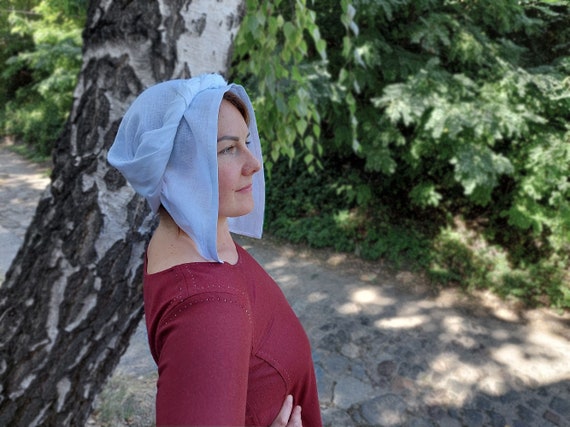This color photograph captures a woman standing in an outdoor, forested setting, facing to the right. She is seen in profile, wearing a dark red (maroon) top and a distinctive blue medieval-style linen bonnet that drapes beneath her chin. Her attire evokes a historical or period dress. She is positioned in front of a tree with striking black and gray bark, characterized by white gaps and deep fissures. Directly behind her, a narrow, grey stone pathway meanders through the forest, dotted with green plants and partially hidden beneath a canopy of tree branches. Sunlight filters through the leaves, casting both light and shadow onto the path, creating a dappled effect on the ground.